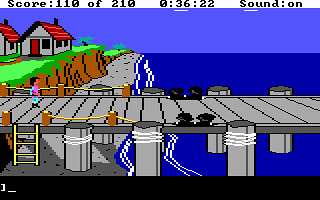This is a pixelated, retro-style 2D video game screenshot. The scene features a little pink-colored character with black hair, teal pants, and black boots, walking to the right along a gray wooden dock. Above, the HUD displays "Score: 110 of 210" and "Sound: On" with a timer at "00:36:22". The background consists of a blue sky and a darker blue ocean. On the left side of the image, a cliff covered in green grass supports gray buildings with red pointed roofs and doors. Hanging off the dock in the bottom left, a yellow ladder is visible. There’s also a small black bar running along the bottom of the image. The entire aesthetic exudes an old-school, simplistic, and pixelated charm.